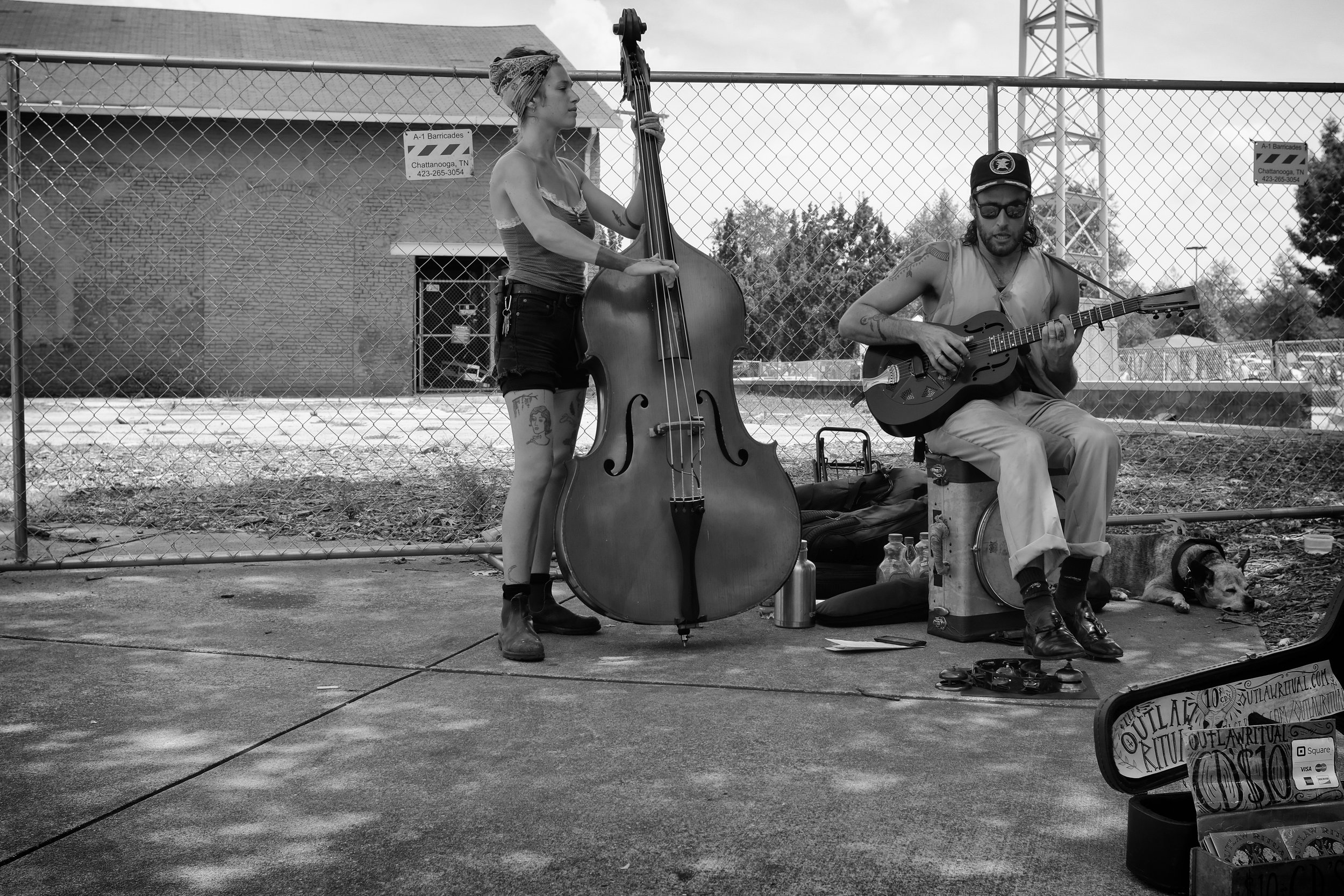In this black-and-white photograph, two heavily tattooed street musicians, a woman and a man, are performing in front of a chain-link fence on a city sidewalk. The woman, approximately 30 years old, stands while playing a large bass guitar with both hands. She wears a tank top, shorts, and a bandana tied in her hair. The man, also about 30, is seated on what appears to be an amplifier and plays an electric guitar. He has long hair, dons a baseball cap with a star on the front, sunglasses, a sleeveless shirt, white pants, and brown shoes. Both are adorned with numerous tattoos. An open guitar case in the lower right corner of the image displays their name, "The Outlaw Ritual", and indicates they are selling cassettes for $10. A dog lies on the ground next to the man, adding to the scene's gritty urban vibe. Behind them, a tall metal structure akin to an antenna rises above the fenced area, which also showcases some trees. The setting suggests an outdoor performance space where people drop tips for their musical entertainment.